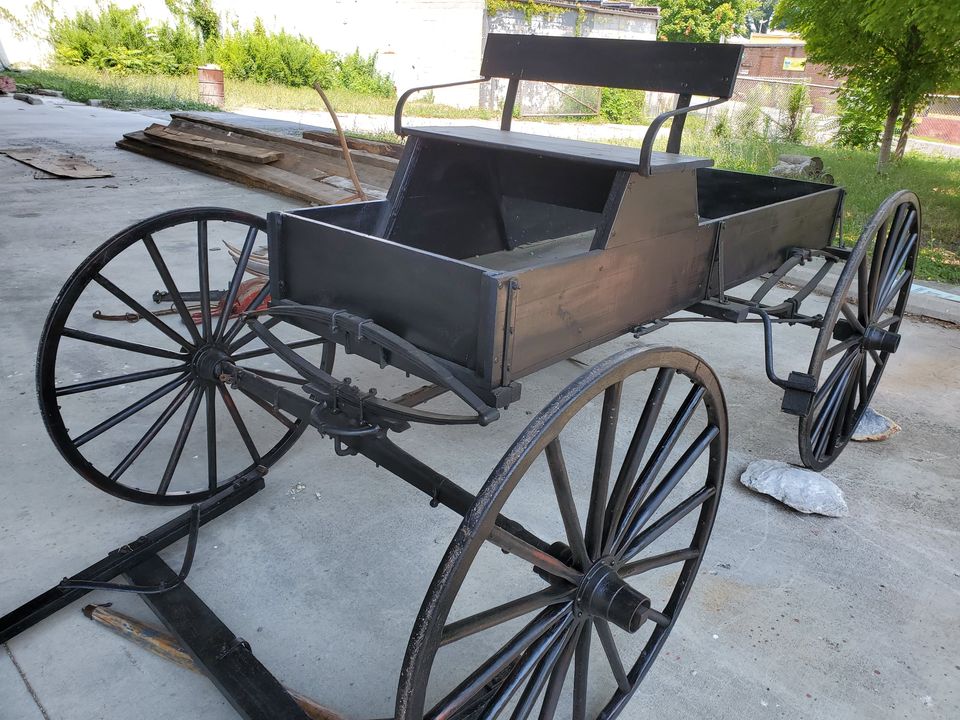The full-color square photograph, taken outdoors during the day under natural but shaded light, features a close-up view of a vintage wooden carriage. The image captures the vehicle on a paved pathway, angled with its front facing slightly leftward and its rear toward the upper right of the frame. The carriage, dark brown in color, showcases its four large spoked wheels, braced against stones to prevent rolling. The design includes a two-person bench seat with a horizontal wooden backrest supported by curved metal arms, and a flat wooden bed, boarded on all sides, meant for carrying supplies or additional passengers.

In the top portion of the photograph, sunlight illuminates part of a white wall, with patches of grass and small plants visible in the upper left corner. To the right, a silver fence encloses a red building, beyond which trees can be seen. The background reveals a mix of grass and the red structure, giving context to the setting—a modern-day display, possibly part of an outdoor historical exhibit. This detailed capture invites reflection on the evolution of transportation from wooden carriages to contemporary modes of travel and beyond.